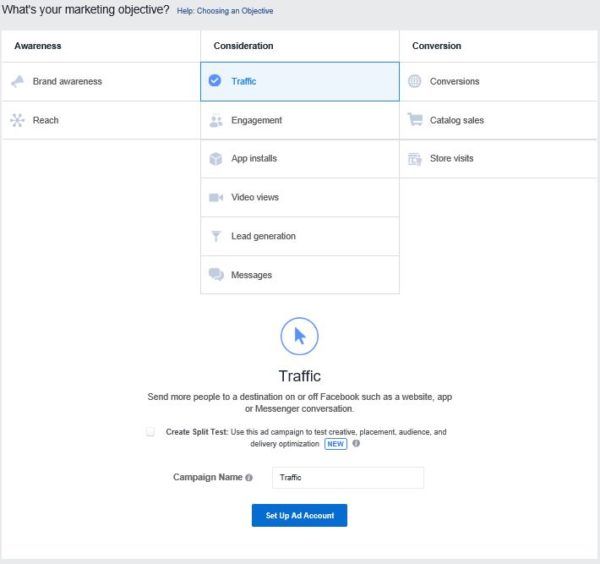The screenshot displays a section titled "What’s Your Marketing Objective?" at the top, set against a gray banner. This section includes a blue clickable phrase, "Help Choosing an Objective." Below this banner, there is a chart divided into three distinct categories: Awareness, Consideration, and Conversion, with each category name presented in bold font.

1. **Awareness:**
   - **Brand Awareness**
   - **Reach**

2. **Consideration:**
   This category features the most options and has the selected objective highlighted in blue with a check mark:
   - **Traffic** (selected)
   - **Engagement**
   - **App Installs**
   - **Video Views**
   - **Lead Generation**
   - **Messages**

3. **Conversion:**
   - **Conversions**
   - **Catalog Sales**
   - **Store Visits**

Under the selected "Traffic" objective, a description details its purpose: "Send more people to the destination on or off Facebook, such as a website, app, or Messenger conversation." An additional option to "Create Split Test" is provided, allowing the user to evaluate the effectiveness of different marketing strategies in driving user actions and connections. The overall layout is designed to assist users in selecting the most suitable objective for their marketing campaigns, emphasizing metrics related to reaching and engaging their target audience and converting leads into tangible business outcomes.